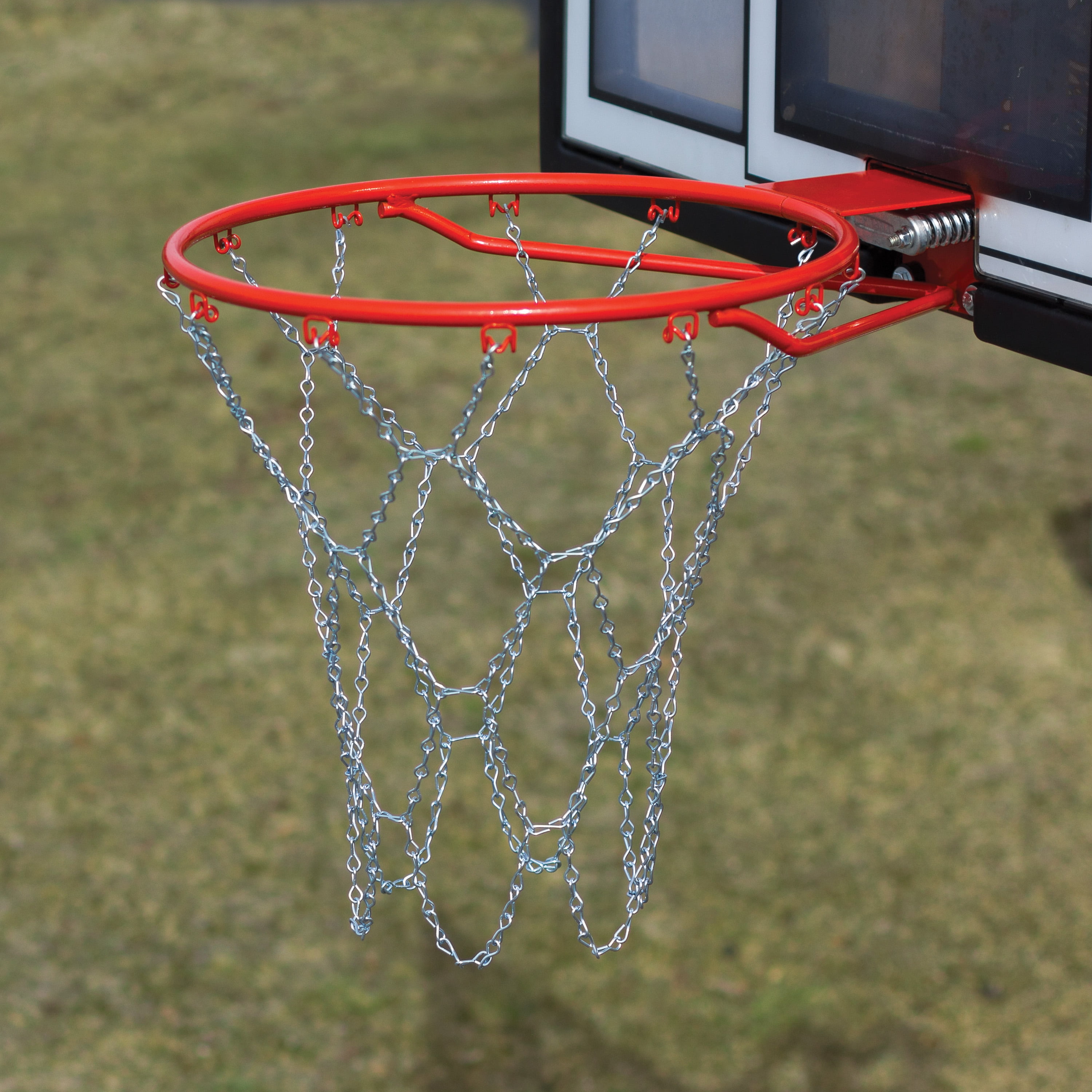The image captures a close-up of a basketball hoop set against a blurred, grassy background, emphasizing the details of the hoop and net. The hoop itself is a bright red rim adorned with a light gray, metallic chain net, which appears brand new and has never been used. The basketball backboard is a rectangular piece made from plexiglass, featuring a distinct black and white color scheme. A small nail or screw is visible, securing the hoop to the backboard. The background is notably out-of-focus, with only vague green and mossy color splotches indicating a grass field, directing full attention to the sharp, contrasting elements of the hoop assembly.